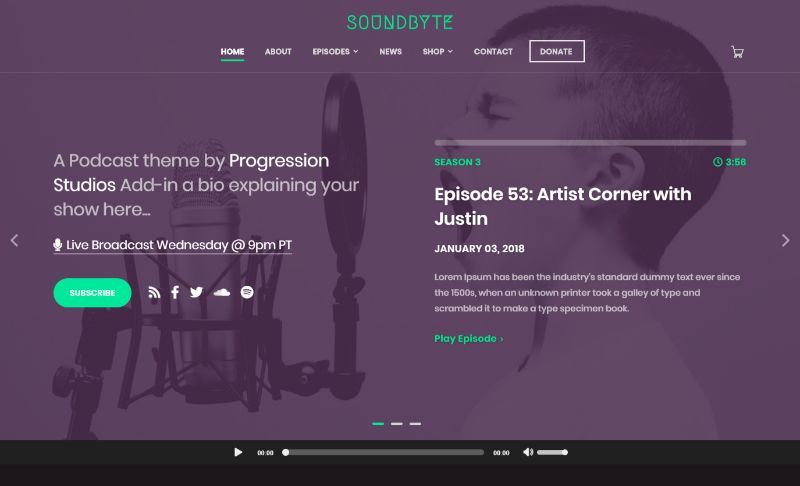This image is a detailed screenshot of the "Soundbite" website. At the top of the page, there are several navigational tabs including Home (currently selected), About, Episodes (with drop-down options), News, Shop (also with a drop-down), Contacts, and a prominent Donate button. A shopping cart icon is visible, indicating the ability to purchase items directly from the site. The website’s design features a purple-toned background with a transparent image of a young boy, sporting a very short haircut, passionately singing or yelling into a microphone.

Prominently displayed on the page is a call to action for listeners: "A podcast theme by Progression Studios. Add in a bio explaining your show here." The site announces a live broadcast scheduled for Wednesdays at 9 p.m. Pacific Time. Visitors are encouraged to subscribe and are provided with links to the show's social media pages.

Additionally, the screenshot highlights a featured episode, "Episode 53: Artist Corner with Justin," which aired on January 3, 2018. This suggests a focus on artistic content and guest features, giving visitors a taste of what to expect from the podcast.